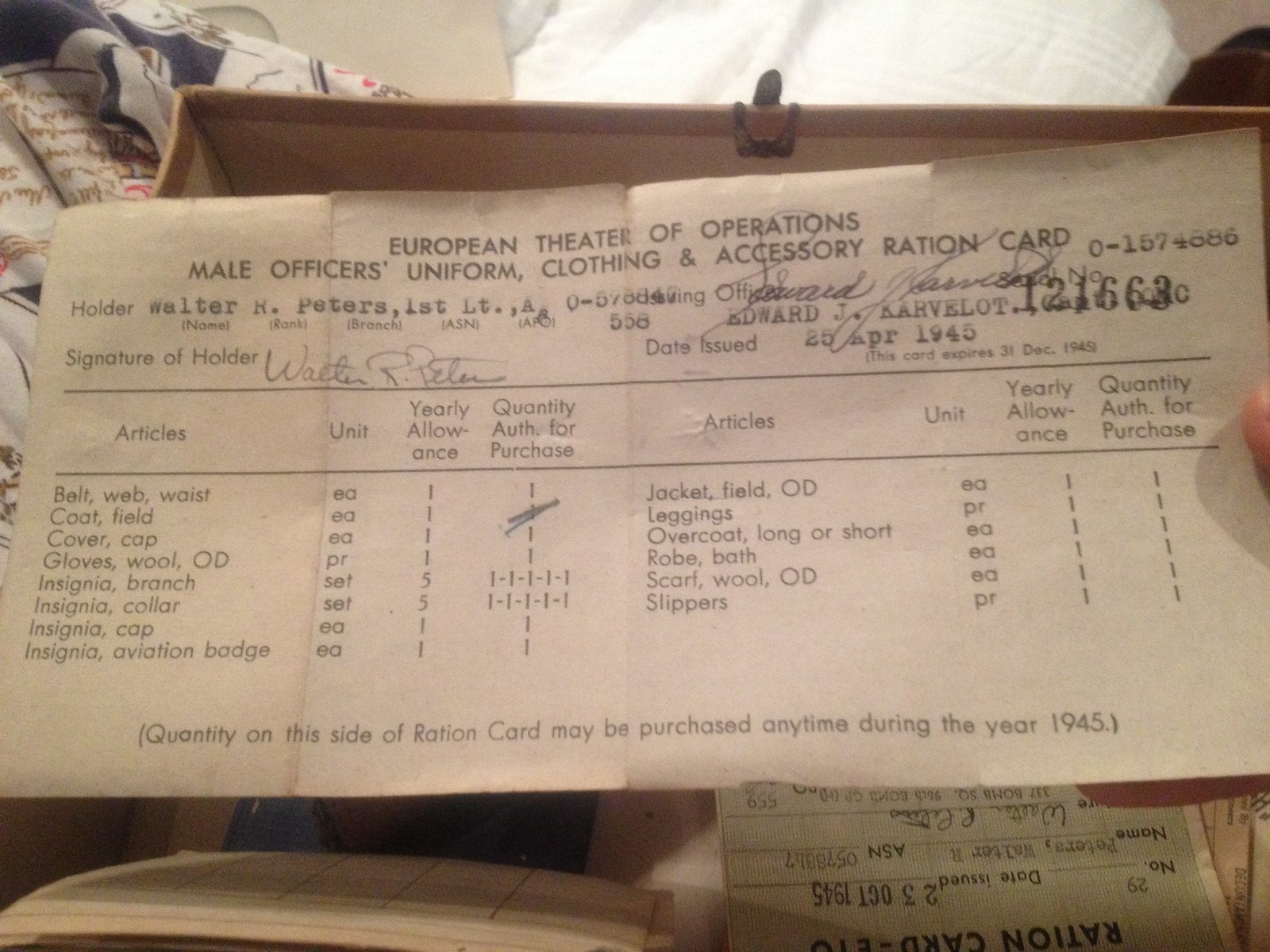This photograph captures a detailed close-up of an aged ration card from 1945, held by the thumb of an unseen person. The primary focus lies on the card's intricate details, prominently bearing the heading "European Theater of Operations, Male Officers Uniform, Clothing, and Accessory Ration Card." Issued on April 25, 1945, this document belonged to First Lieutenant Walter H. Peters. The card includes an official stamp numbered 121663 and contains Peters' signature. Below the header, a meticulously itemized table lists various articles such as belts, coats, caps, insignia sets, jackets, overcoats, scarves, slippers, and more, detailing the unit, yearly allowance, and quantity authorized for purchase. The text at the bottom specifies that items could be purchased anytime within the year 1945. The background of the image reveals a box filled with additional documents and another partially visible ration card, reinforcing the historical and archival nature of this keepsake. The photograph is rendered in a monochromatic palette of black, white, gray, blue, green, brown, and peach tones, emphasizing the vintage essence of the scene.